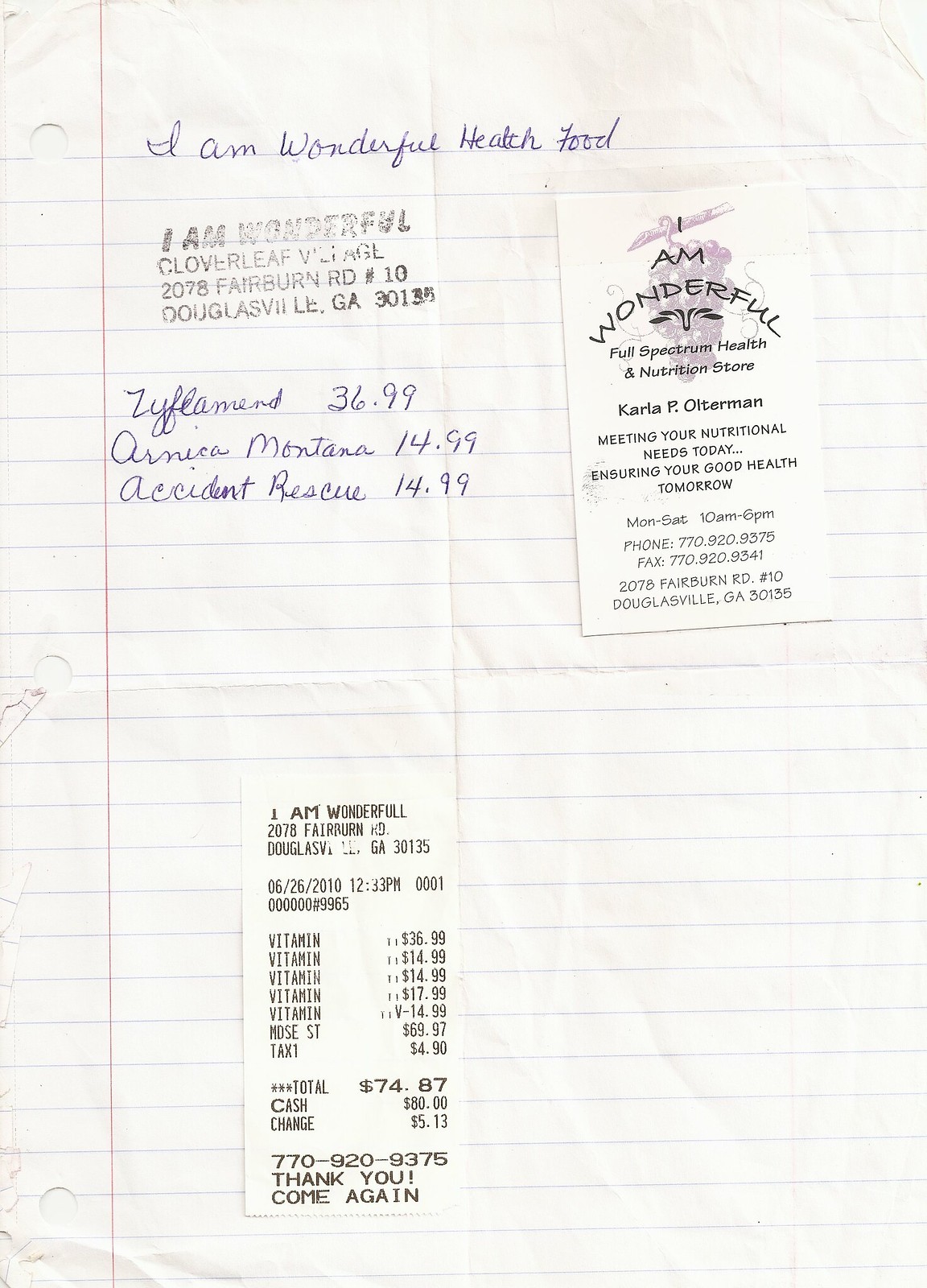This photograph features a collection of documents that appear to have been copied, each providing unique details related to a health food business. 

The first document is a piece of notebook paper, handwritten in pen. At the top, it declares, "I am wonderful health food," followed by an address for a business located in Douglasville, Georgia. Below this heading, there are several items listed in cursive handwriting, each accompanied by a price: $36.99, $14.99, and $14.99.

On top of the notebook paper are two additional documents. The first is a receipt that itemizes various vitamins purchased, with a total amount of $74.87. The final item is a business card bearing the name Carla P. Otterman, suggesting an affiliation with a health food business.

Overall, this detailed photograph provides insight into a health food enterprise located in Douglasville, Georgia, highlighting specific items, prices, and personnel associated with the business.